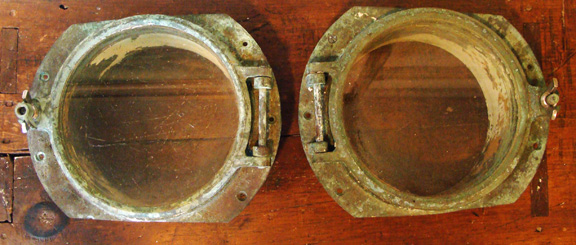The image depicts two old, circular metal objects that resemble porthole covers, laid on a worn-out, wooden table. The objects are heavy-looking, rusted, and exhibit a brownish color indicative of decay, suggesting they have possibly been exposed to water for an extended period. The one on the left is slightly smaller and lighter in color, while the one on the right appears dirtier and more rusted. Both items have hinges on one side, implying that they could be opened, although it's unclear if there's any glass involved. The horizontal photo showcases these objects in a rectangular frame, with the table's surface visible through the rings.